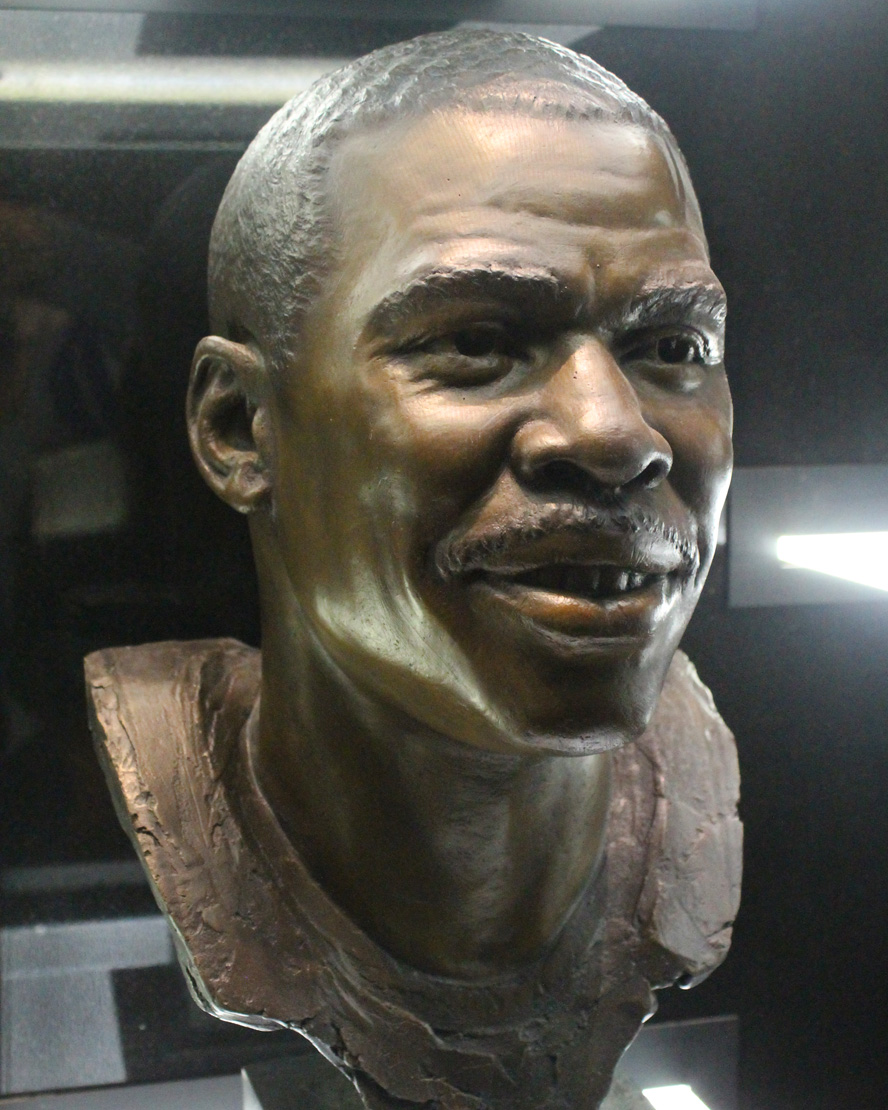The image captures a color photograph in portrait orientation, showcasing a bronze sculpture of an African-American man's head and neck. The sculpture radiates a lifelike presence, characterized by its golden bronze hue and somewhat reflective finish. The man’s face is depicted with a full smile, exuding confidence and warmth, and he is gazing slightly upwards to the right side of the image. His features include very short hair, a furrowed brow, and large bushy eyebrows. The bronze extends around the neck in an irregular shape, resembling a collar, marking the end of the sculpture. The display setting appears to be indoor, potentially an exhibition or museum, with an overall dark ambiance softened by overhead lighting that highlights the details of the statue. The background is composed of indiscernible dark and chrome rectangular shapes, adding to the refined, realistic essence of the photograph, which falls under the style of photographic representational realism.